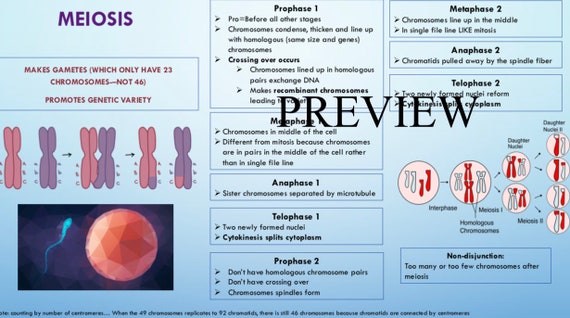This image is likely from a textbook or guidebook illustrating the scientific process of meiosis. It has a light blue background and is divided into three columns. In the top left corner, bold purple letters spell "MEIOSIS." Below this, red text reads "Makes gametes, which only have 23 chromosomes, not 46," followed by "Promotes genetic variety." A sketch of paired chromosomes in pink and purple follows this text, and beneath it, there is a drawing of a pink egg cell with a blue sperm cell nearby on the left.

The right side of the image is segmented to detail the stages of meiosis, including prophase 1, anaphase 1, telophase, and anaphase. Each section includes descriptive text, and in the final section, telophase 2, there are graphics and drawings showing different chromosomes. Black text across the middle and right columns states "Preview," echoing the instructional nature of the visual content.